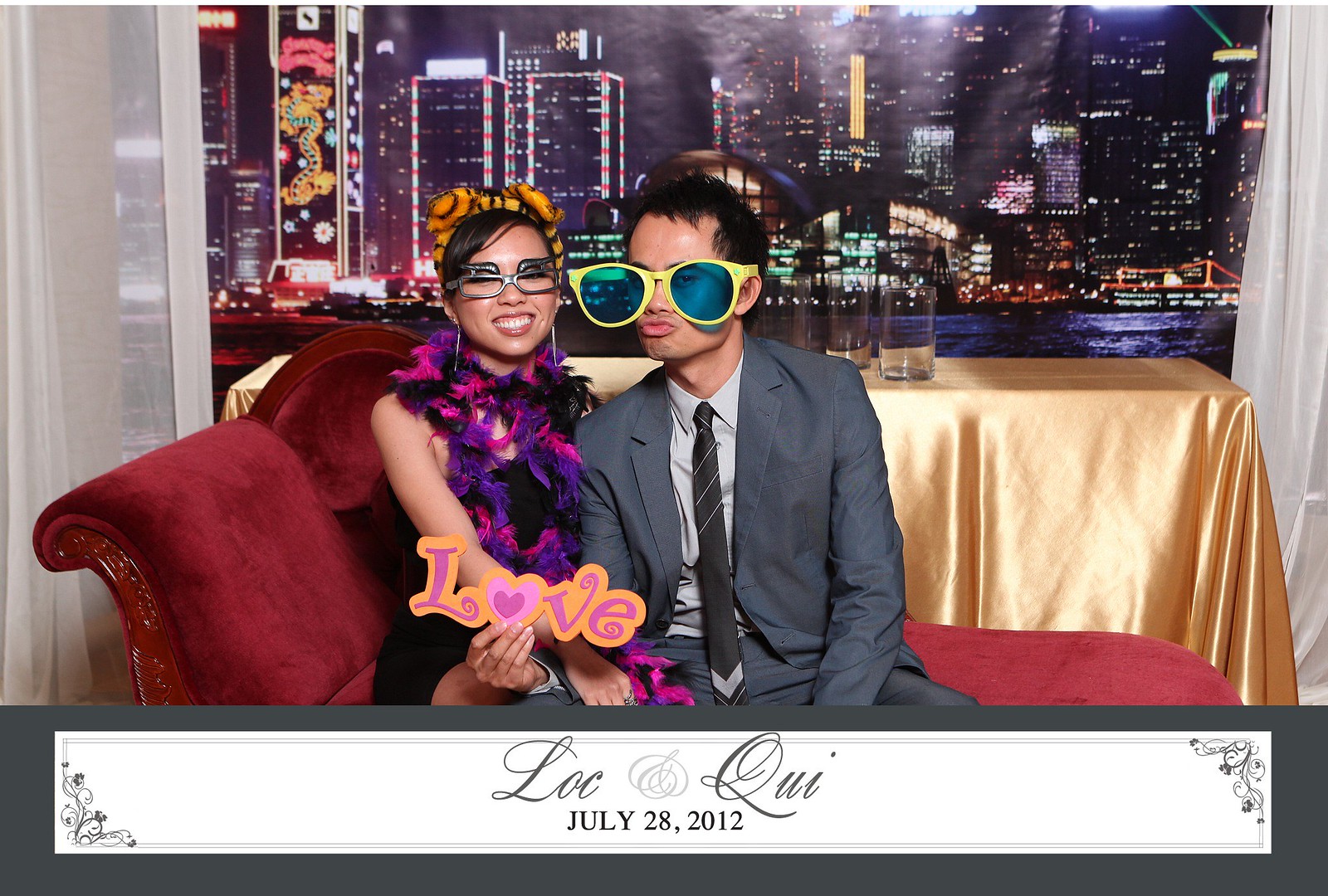In this comedic and whimsical photograph, two people are seated on a vintage red sofa in front of a table adorned with a gold tablecloth, which holds a few glasses or vases. Behind them, an expansive window reveals a vibrant cityscape, illuminated with various nighttime lights. The man on the right, dressed in a gray suit with a black tie, is making a puckering face while sporting hilariously large yellow-framed sunglasses with blue lenses. He holds a cutout sign reading "LOVE," where the 'O' is heart-shaped, in pink and orange colors. Seated next to him is a woman wearing a black dress accessorized with a multicolored pink, purple, and black scarf, tiger ear headband, and glasses with exaggerated eyebrows. Below them, the caption reads "Loke and Uwe, July 28th, 2012," capturing the playful essence of the moment.